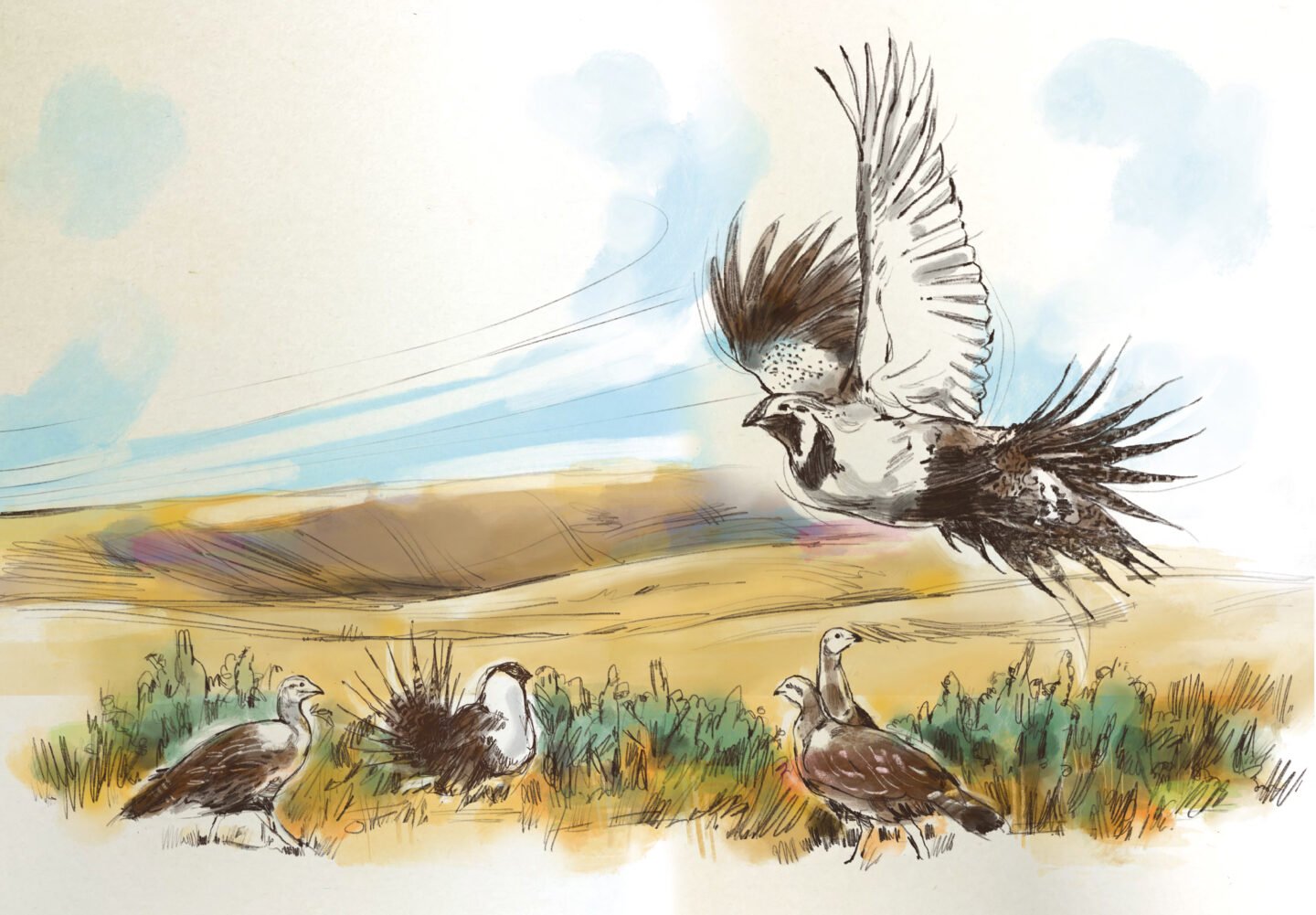The vibrant sketch depicts a field scene with multiple birds. In the foreground, several birds are positioned among tufts of grass with green tops, offering the most detailed element against the broader tan expanse of the field that extends into a distant ridge. The sky, which occupies the upper half of the image, is partly cloudy with streaks of blue and suggests a bright daylight ambiance. Notably, there are four birds on the ground, all possessing brown wings and white undersides, suggestive of a species resembling grouse. Each bird has distinct brown and white patterns on its face and body, with spots on their backs. Among the grounded birds, one stands out with a wild tail pattern and poofy white areas on its face and chest. Above this scene, a single bird with the same brown-and-white coloration soars gracefully, emphasizing the dynamic composition of the image. The distant low mountain range adds depth to the background with its tan, brown, and white tones, contributing to the painted, naturalistic quality of the artwork.